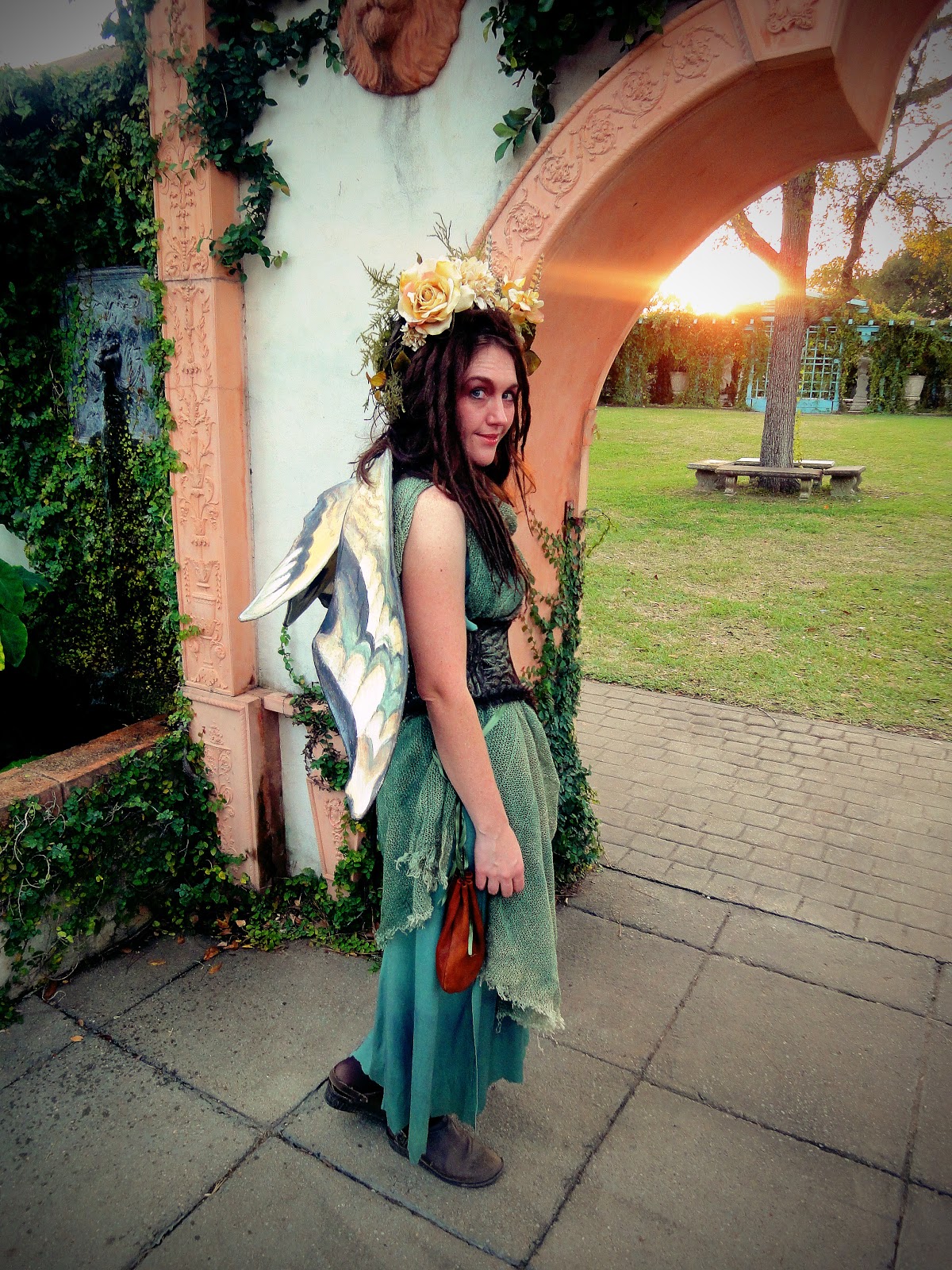In the image, a woman dressed in an elaborate fantasy Renaissance costume is standing under an ornate archway. She has long brown hair and her head is turned towards the camera, smiling with her right shoulder facing it. Her outfit features fairy wings, a green and blue ragged skirt, a black corset, dark brown boots, and a leather satchel. A standout accessory is the large flower crown on her head composed of cream or peach-colored roses.

The archway itself is intricate, crafted from light pink bricks with ornate scrollwork and a white relief sculpture at the top, possibly depicting a lion. Ivy and vines climb up the structure, adding to the old-world charm. Beyond the archway, the scene opens up to what appears to be a garden or courtyard. There is a blue building with numerous small glass windows, a tree with a circular bench, and neatly trimmed grass. The sun is setting in the background, casting a warm, gentle glow over the scene. The woman is standing on a concrete floor that transitions into a paved and brick sidewalk.